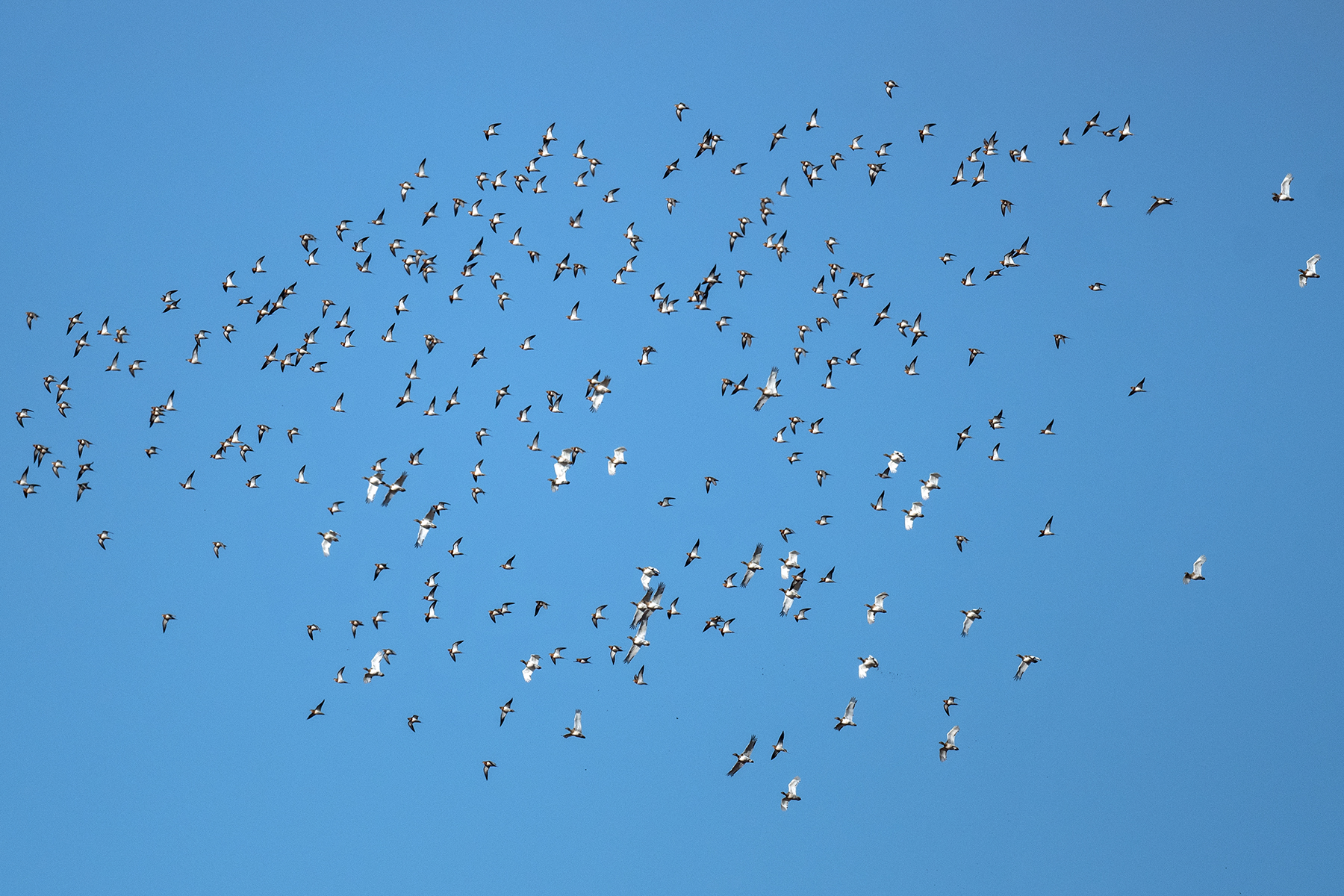The image captures a large flock of birds soaring through a clear, nondescript blue sky during the daytime, illuminated by sunlight. The birds, with white undersides to their wings and dark-colored bodies and beaks, are scattered throughout the sky, appearing mostly as shadowed silhouettes. While the majority of the flock moves from left to right, a few birds fly in opposite directions, suggesting a circular motion as if searching for something below. Some birds fly densely clustered in the center, while others are more solitary, particularly one bird noticeably distant from the group. The specific type of birds is indistinguishable due to their small size and distance.